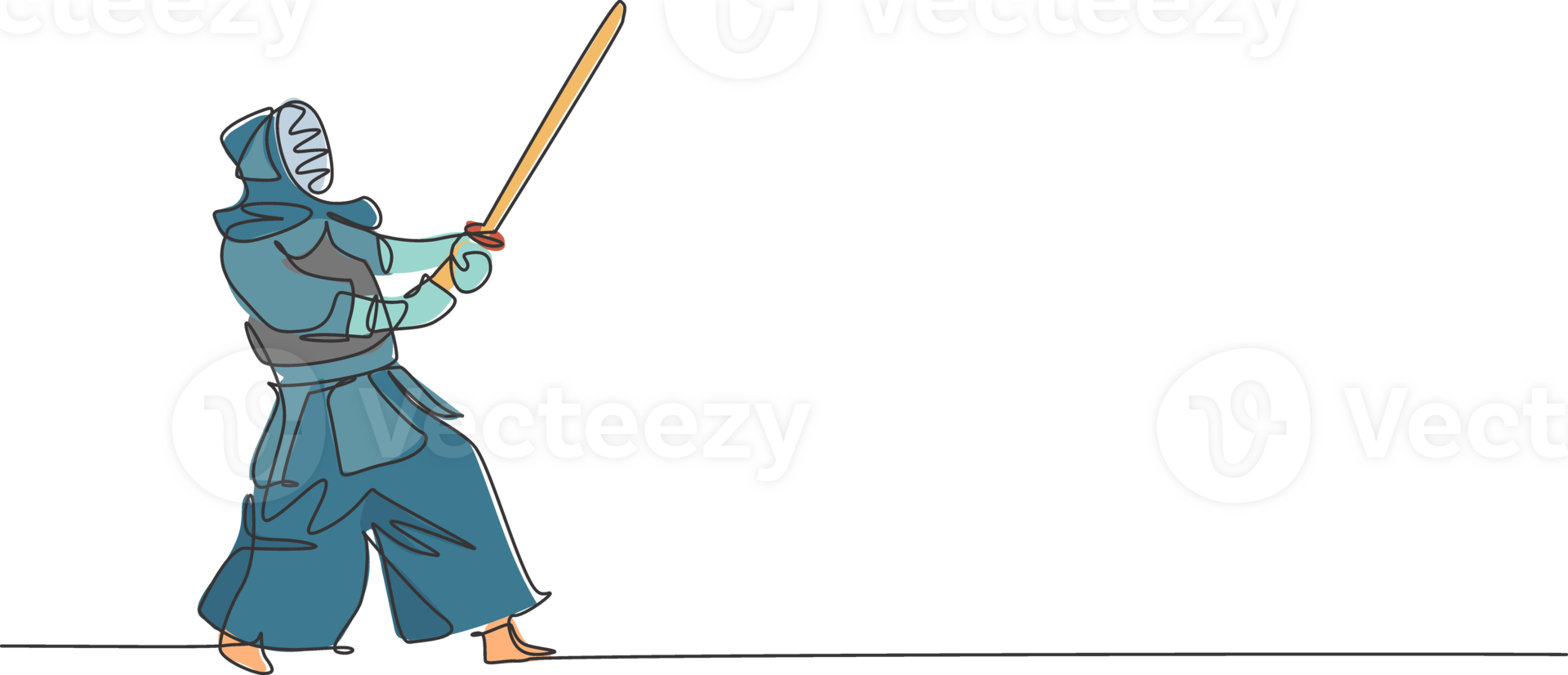The image depicts a hand-drawn, horizontally rectangular cartoon of a warrior standing on the left side with a minimalist black line along the bottom. The background of the image is white with a semi-faded watermark running throughout, repeatedly displaying the text "V-E-C-T-E-E-Z-Y." The warrior is illustrated with striking detail: he is dressed in a traditional blue and gray outfit resembling a samurai's garb, but he sports a fencer's mask covering his face for added protection. His uniform consists of a blue jacket, billowy blue pants that taper at the ankles, turquoise blue gloves, and a gray chest piece that serves as light armor. His feet are bare, and he holds a wooden samurai-style sword, distinguished by its brown blade and red hilt. The character's outline is crafted with a single continuous black line, giving a cohesive flow to his form. He appears to be in a ready stance, poised for action against a stark, white backdrop.